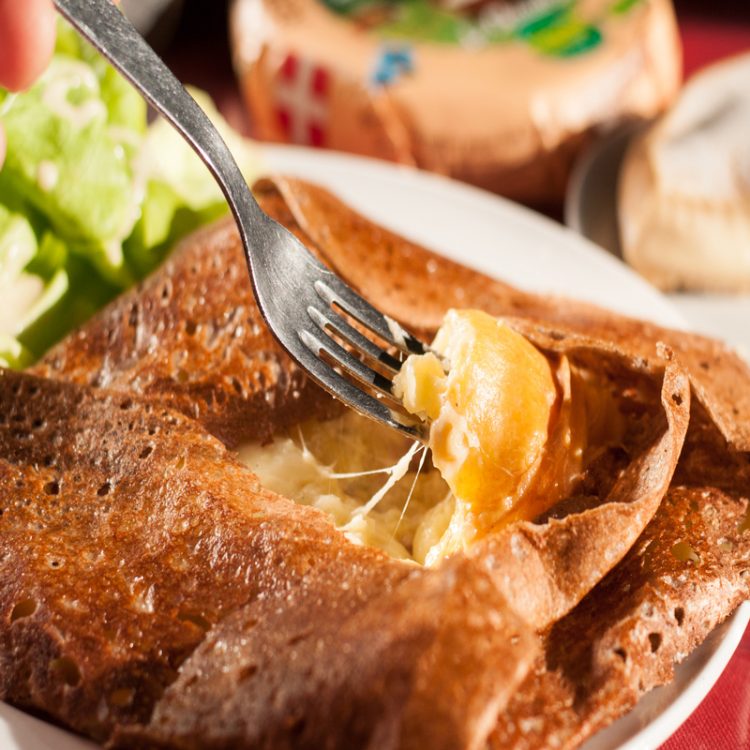This color photograph, shot in a square format, features a close-up view of a delectable food scene set indoors. At the forefront is a beautifully baked pastry, likely a fruit galette, on a pristine white china plate. The galette has a golden-brown, folded-over crust with a central opening revealing a tantalizing filling, accented by an orange hue, possibly containing fruit and strings of melted cheese. A silver fork, marred with a few scratches, pierces this filling, lifting a piece out of the pastry and drawing the viewer’s eye to the intricate textures and colors.

In the background, to the upper left, there is a hint of green, which appears to be avocado or a small salad, adding a fresh contrast to the scene. Further back, slightly out of focus, rests a cake adorned with red and white cross decorations and embellished with orange and green frosting. Adjacent to the cake, another pastry or food item can be seen on a silver platter. The setting is completed by a vibrant red tablecloth that underlines the plate, enhancing the warm tones of the entire composition. The photograph is a detailed representation of food in a realistic style, capturing the essence of an inviting and meticulously arranged meal.